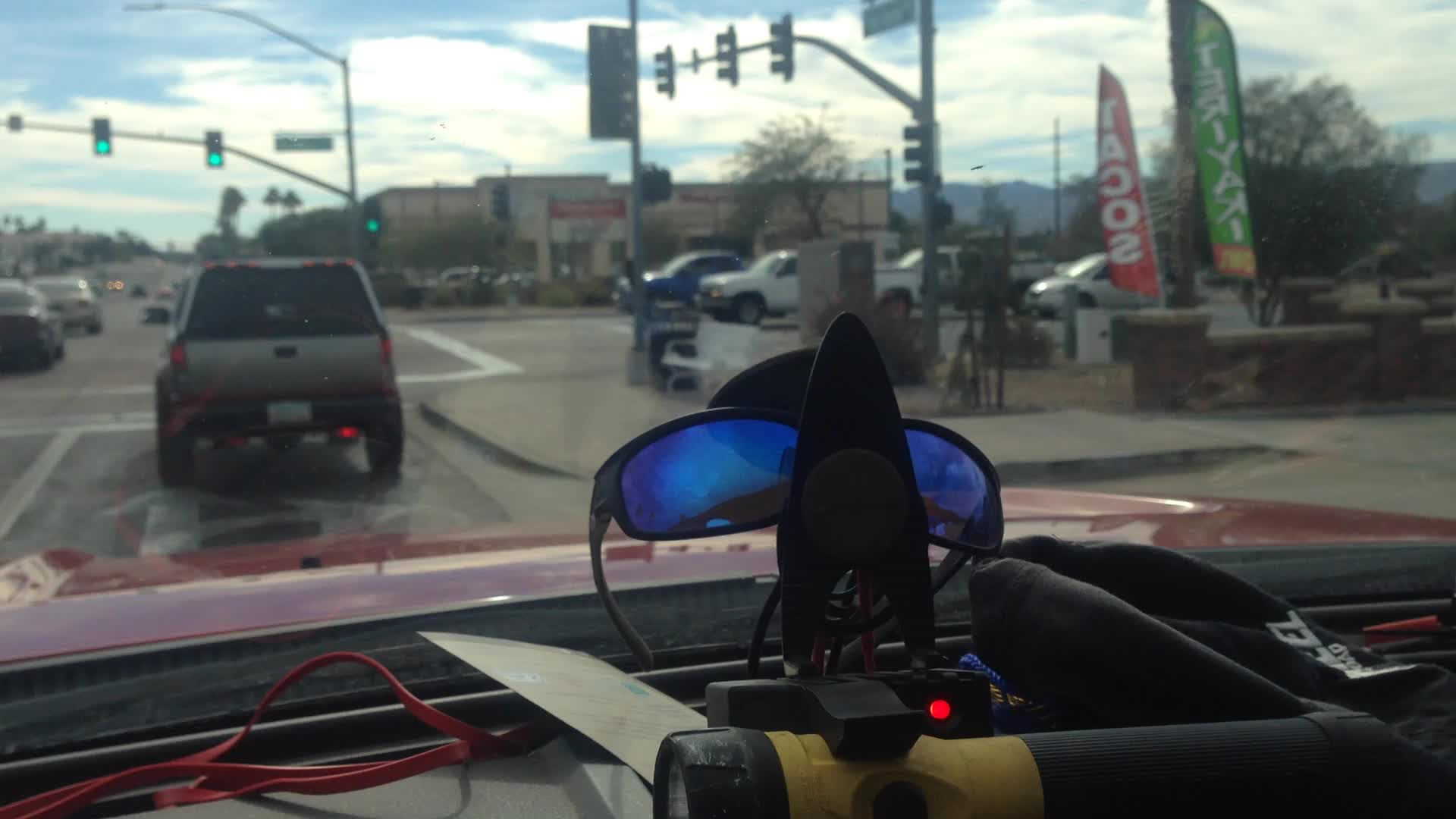The image captures the front section of a car's interior, focusing prominently on the top of the dashboard. A pair of sunglasses with bluish-tinted lenses and black plastic rims, looking perfect for a beach outing, sit in an upward-facing holder. The holder itself is elongated and triangular, tapering to a circular end. Beside the sunglasses, a yellow and black flashlight is visible, easily identifiable by its black handle. Additionally, there is an ID card resting on the dashboard. Through the windshield, an urban cityscape is visible in the background, providing context to the setting.